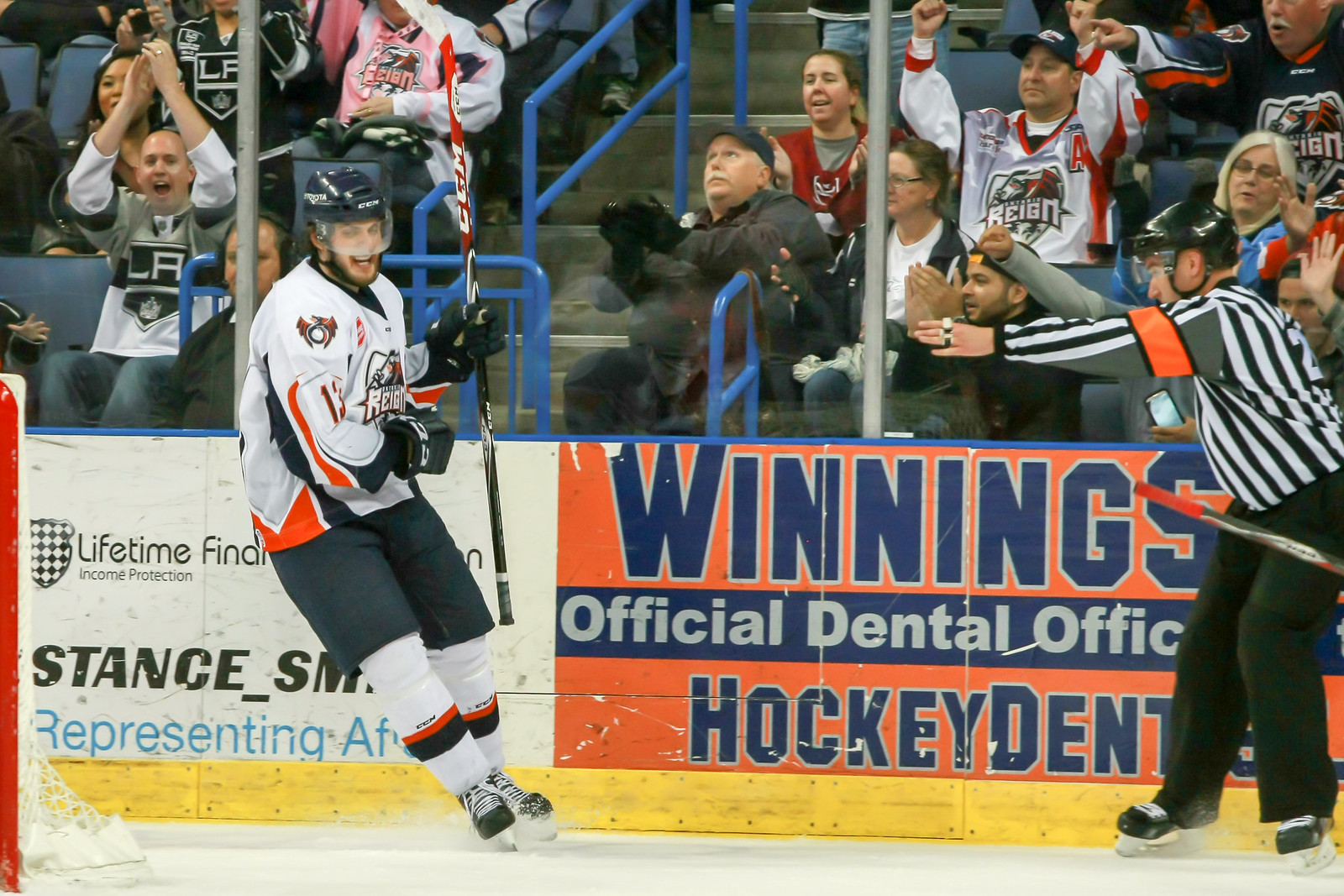In this detailed image of an indoor hockey game, the scene is set on a pristine ice rink. Dominating the center of the image is a triumphant hockey player, apparently celebrating a goal. He is dressed in a white, orange, and blue jersey, black shorts, white socks, black skates, and protective gear including a black helmet and gloves. He holds his stick aloft in a victory pose and leans slightly to his right. To the far right of the image stands a referee in the characteristic black and white striped uniform with black pants and an orange band around his upper left arm.

Behind the main action, the background features a high wall with glass panes. Beyond the glass, several rows of enthusiastic spectators can be seen, some of whom are clapping and wearing jerseys similar to the player on the ice. These fans add to the celebratory atmosphere.

Visible on the boards by the ice are advertisements. One prominent sign displays the text "Wennings Official Dental Office, Hockey Dental" while another nearby sign reads "Lifetime Income Protection," though portions of the text are obscured by the player's legs.

The image palette includes vibrant colors such as red, white, black, blue, yellow, orange, gray, maroon, and pink, contributing to the lively and dynamic ambiance of the scene. The overall setting suggests an active, indoor hockey game, though the time of day remains indeterminable.